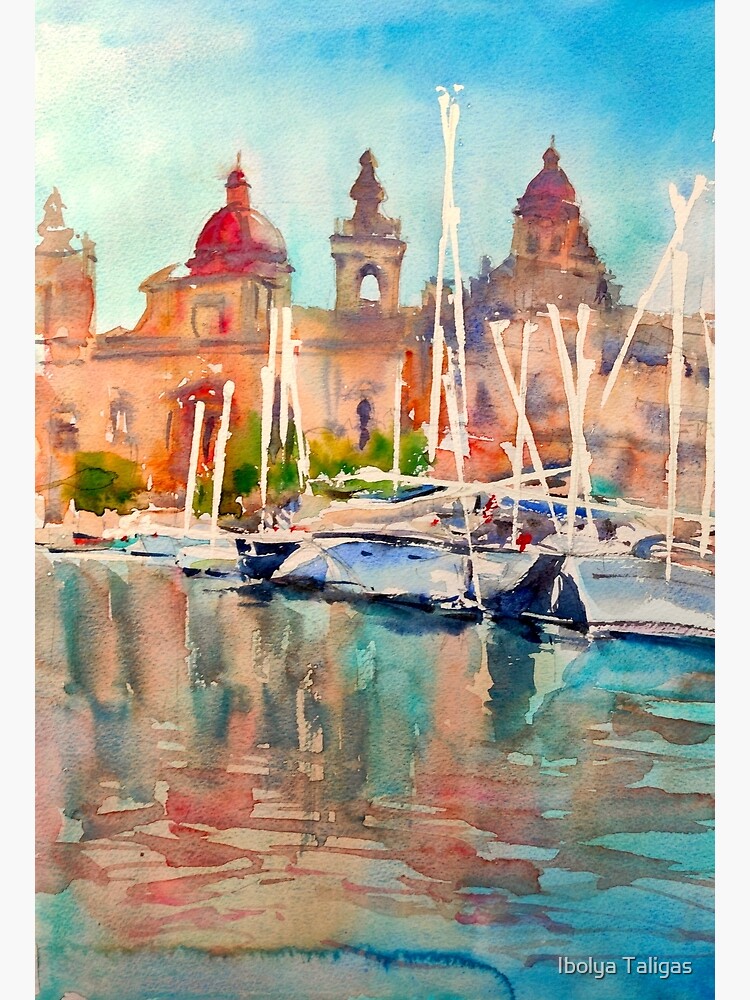This painting, reminiscent of an impressionist style with watercolor-like qualities, depicts a serene bay scene. In the foreground, a tranquil body of water reflects the myriad hues of the surroundings—shades of blue, pink, and tan. Nestled on the water are sailboats, predominantly whitish-blue in color, with their tall, white masts standing bare against the sky. The boats seem to point upwards, their reflections dancing on the water's surface.

Behind the boats, the painting transitions to a harbor area adorned with an array of structures. These buildings, rendered in a blend of reds, browns, pinks, oranges, and greens, showcase various architectural elements such as domes, steeples, and towers. One prominent building features a tower with an arch, while another on the right is marked by a tall dome. The sky above is a calming light blue interspersed with sporadic white clouds.

All these elements blur softly into each other, creating a dreamlike and abstract representation of the scene. In the bottom right corner, the artist’s signature, "Ebolia Taligas," is distinctly marked.